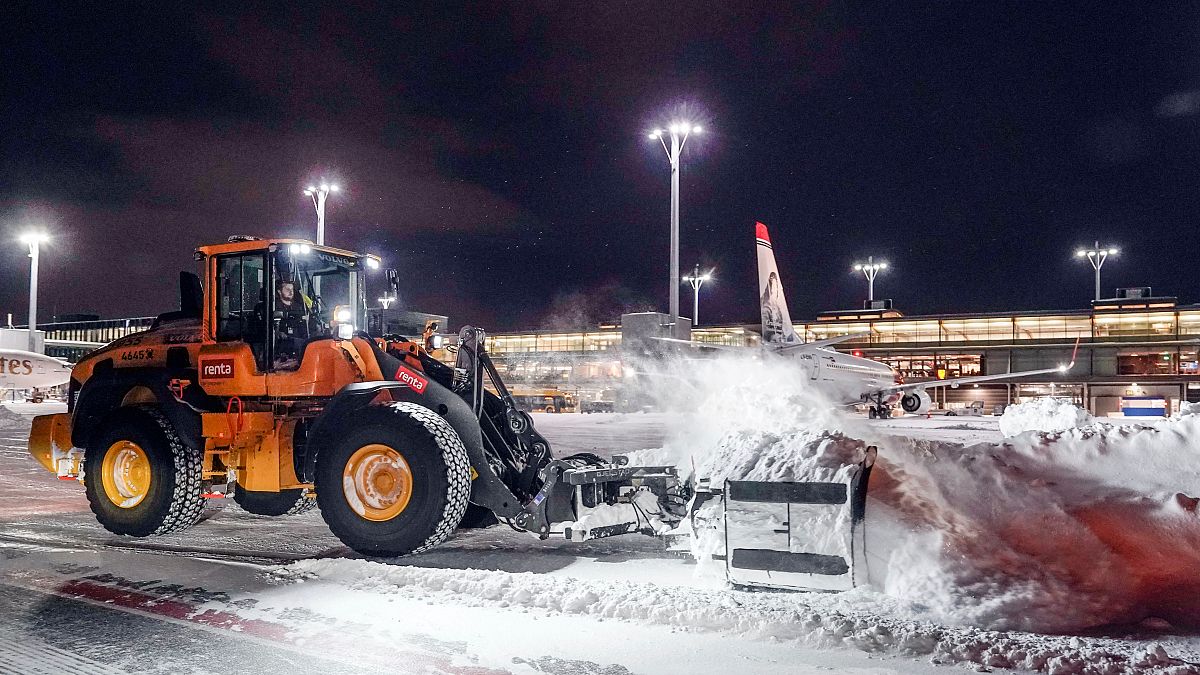This nighttime photograph captures a scene at an airport blanketed in snow. Dominating the foreground is a vibrant orange and black tractor, equipped with a snowplow attachment, diligently clearing snow from the runway. Powerful floodlights illuminate the area, casting a stark contrast against the dark night sky and accentuating the snow-covered ground. In the background, several aeroplanes are faintly visible, lined up and awaiting their turn for departure or arrival. A solitary figure, presumably an airport worker, is at the helm of the tractor, steering it with precision to ensure the runway remains navigable. Beneath the freshly cleared snow, the dark gray markings of the runway become discernible, hinting at the meticulous effort taken to keep the airport operations smooth despite the wintry conditions.